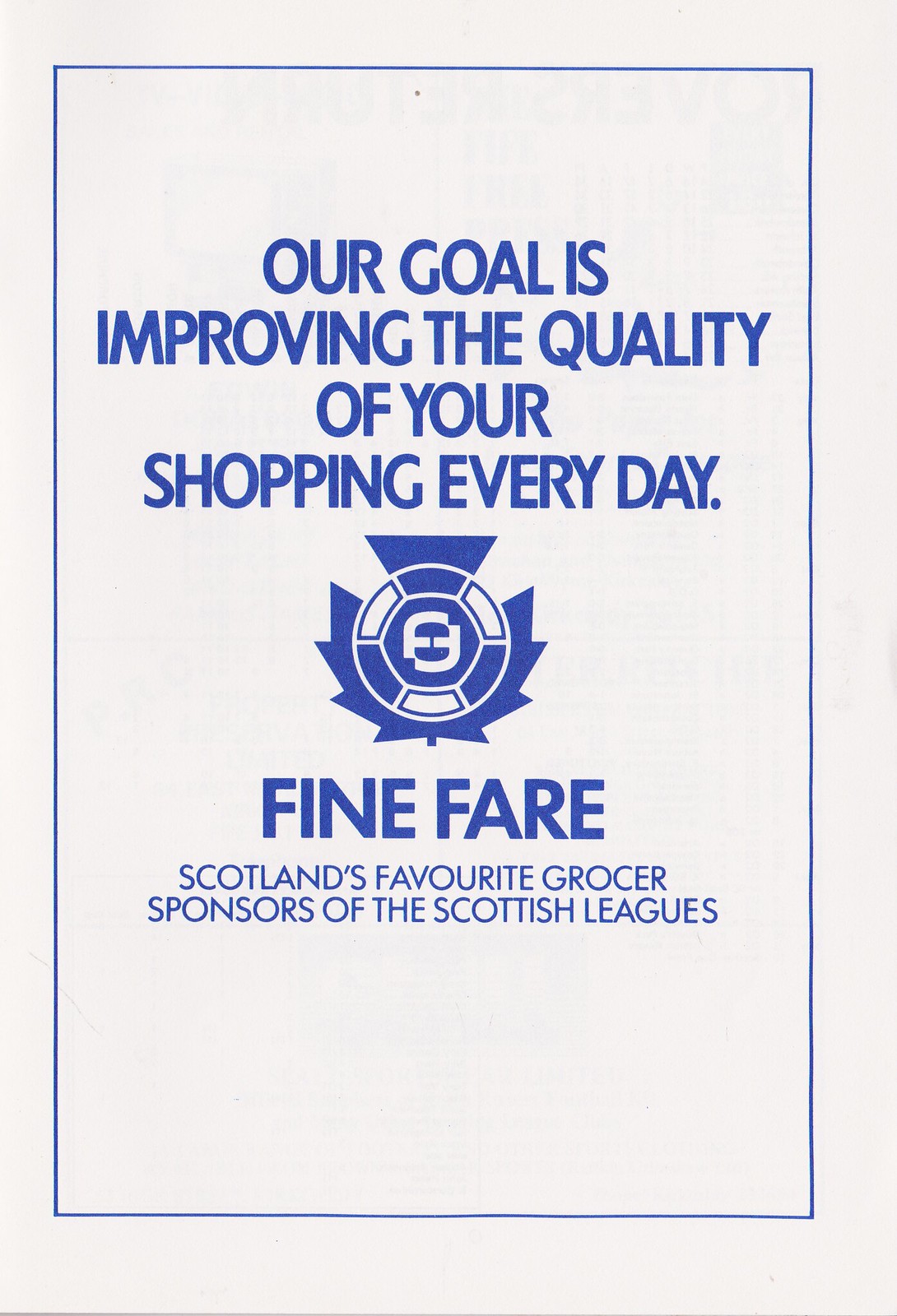This image features a tall, rectangular advertisement poster with an off-white background. Encased within a dark blue, rectangular border, the text inside is also in dark blue. At the top, bold and in all capital letters, it reads: "OUR GOAL IS IMPROVING THE QUALITY OF YOUR SHOPPING EVERY DAY." Below this, there is a logo resembling a blue and white soccer ball superimposed on a blue maple leaf. Beneath the logo, bold text reads "FINE FAIR," followed by smaller, less bold text that states "Scotland's Favourite Grocer" and "Sponsors of the Scottish Leagues." This detailed advertisement emphasizes the grocery store's commitment to enhancing the shopping experience while highlighting their sponsorship of Scottish football leagues.